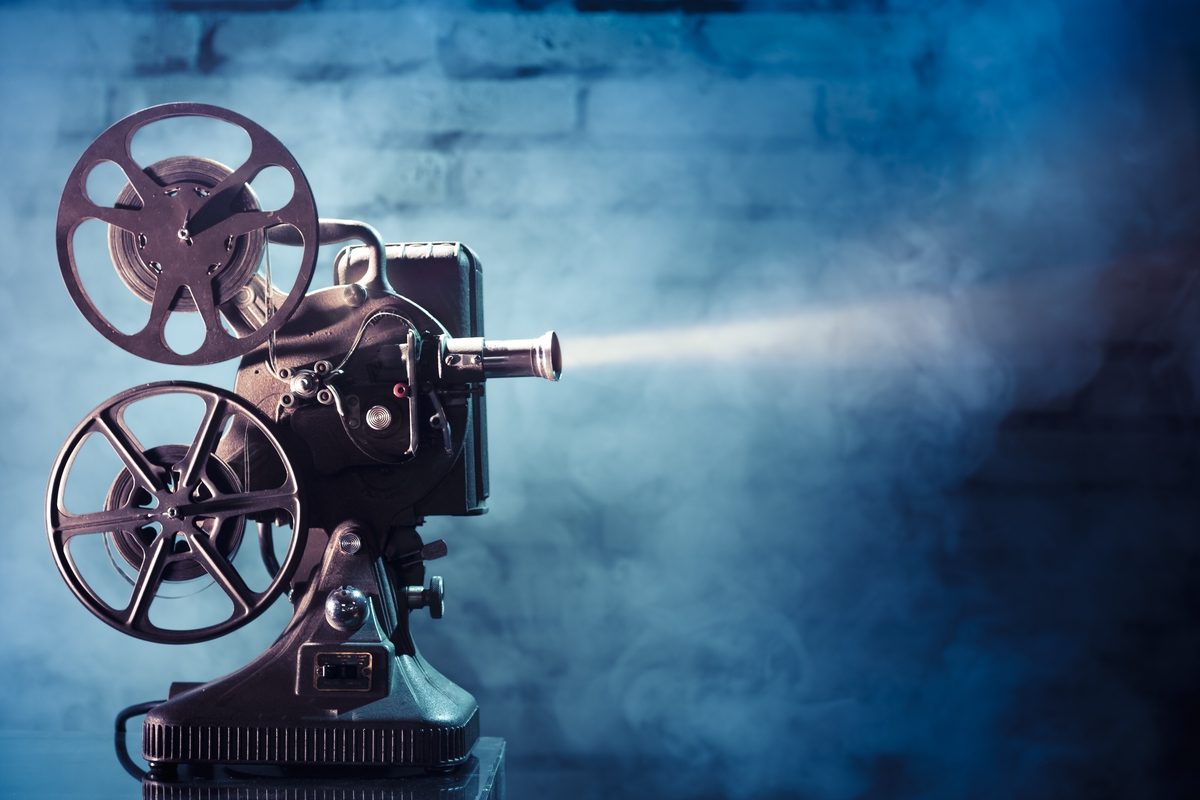The image depicts an old-fashioned black film projector positioned on a table in a dimly lit, ominous room. The projector, seen in profile and pointing to the right, lacks film reels but is switched on, casting a beam of light through the foggy atmosphere. The room, reminiscent of a crypt or tomb, is characterized by its brick walls and a bluish haze that accentuates the eerie ambiance. Despite the absence of film, the projector appears to be in clean and good condition, adding a stark contrast to the otherwise dingy and skeletal surroundings that look like a setting right out of a horror movie.